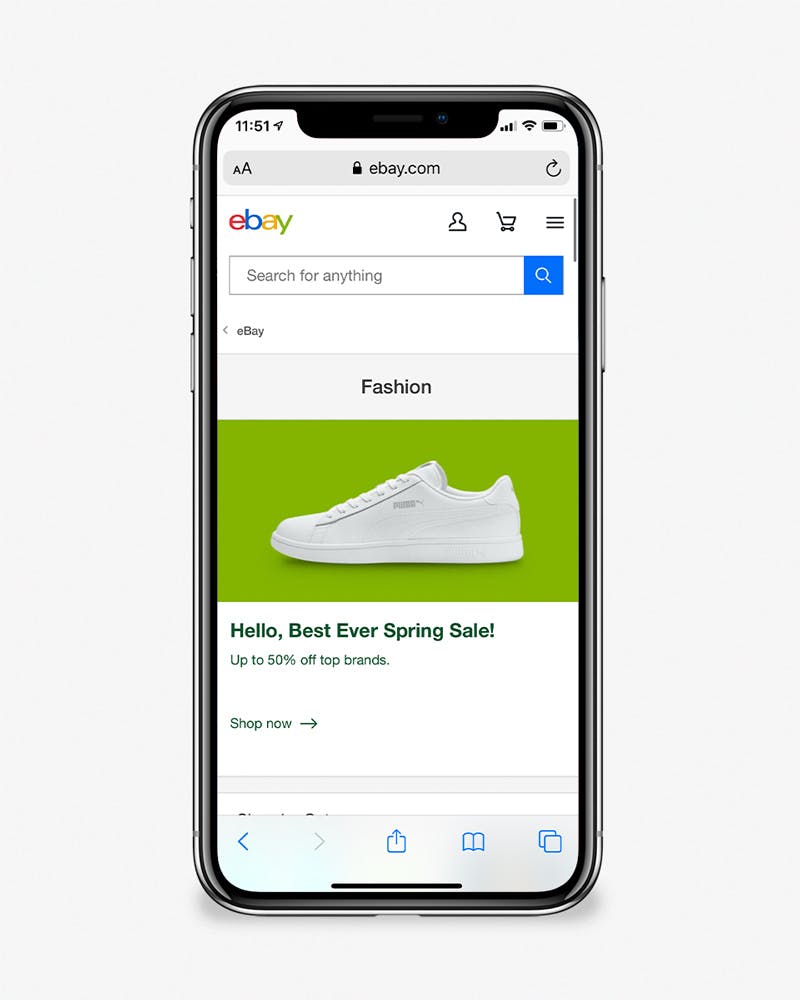The image showcases an Apple iPhone displaying the eBay website. The screen is focused on the Fashion category, highlighted by a lime green bar beneath the category name. Centered on the screen is an image of an all-white low-top leather Puma sneaker, likely categorized under women's fashion athletic shoes. Below the sneaker image, there is a promotional text stating, "Hello, Best Ever Spring Sale - Up to 50% off Top Brands." Further down, a "Shop Now" button is clearly visible, inviting users to explore more spring items available at up to 50% off.